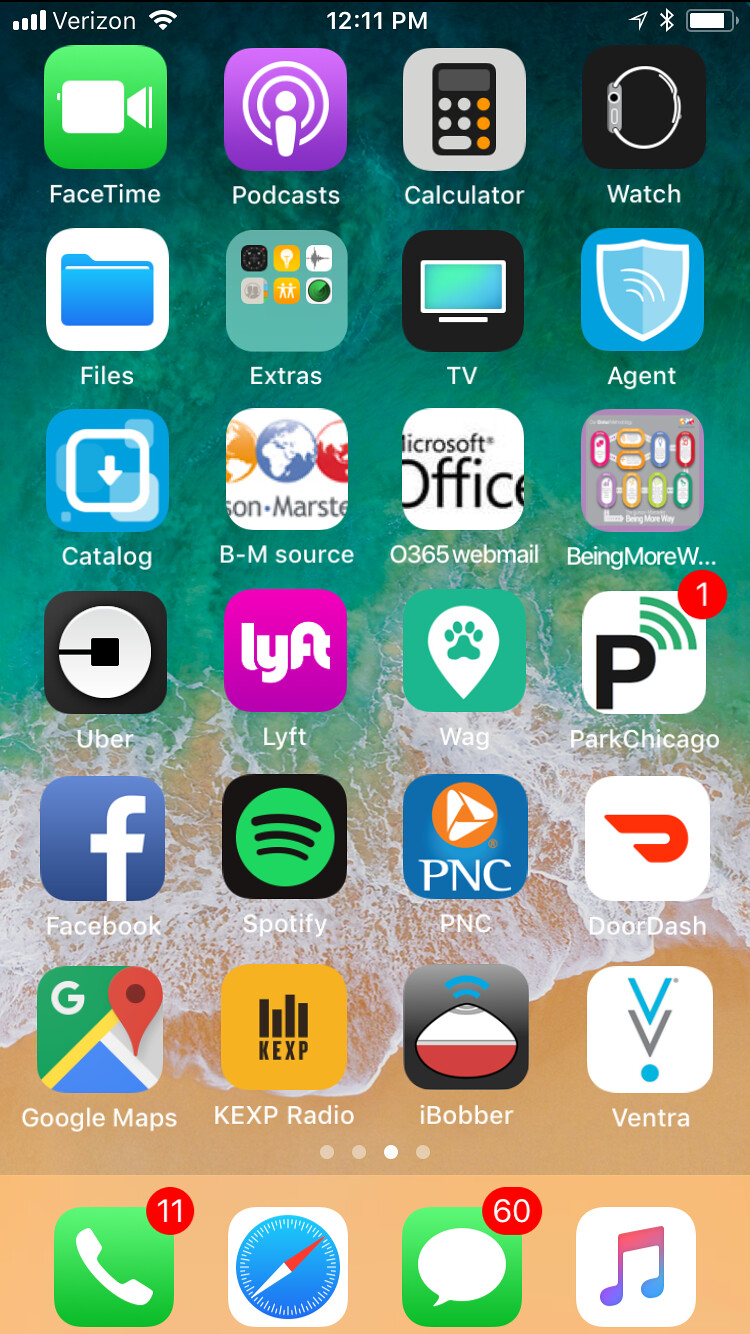The image showcases a smartphone screen with a detailed interface. At the top, it displays standard indicators: a strong signal reading "Verizon," Wi-Fi connectivity, the time - 12:11 p.m., an active Bluetooth connection, and a battery indicator. Below, the screen is filled with numerous app icons against a serene greenish-blue water background that transitions to sand at the bottom.

The upper portion reveals the user has pending 11 phone messages and 60 text messages. Below, four fixed icons are positioned at the bottom row, presumably for essential apps. Scattered across the screen are various app icons including FaceTime, Podcast, Calculator, Watch, Files, Extra, 365 Webmail, Park Chicago, WAG, Lyft, Uber, Facebook, Spotify, PNC, DoorDash, Google Maps, KEXP Radio, iBobber, and Ventra.

Despite the high number of visible notifications, there are no email alerts, highlighting a notable absence of email activity. The meticulous arrangement of icons fully occupies the screen, maximizing space while emphasizing the aquatic-themed background.